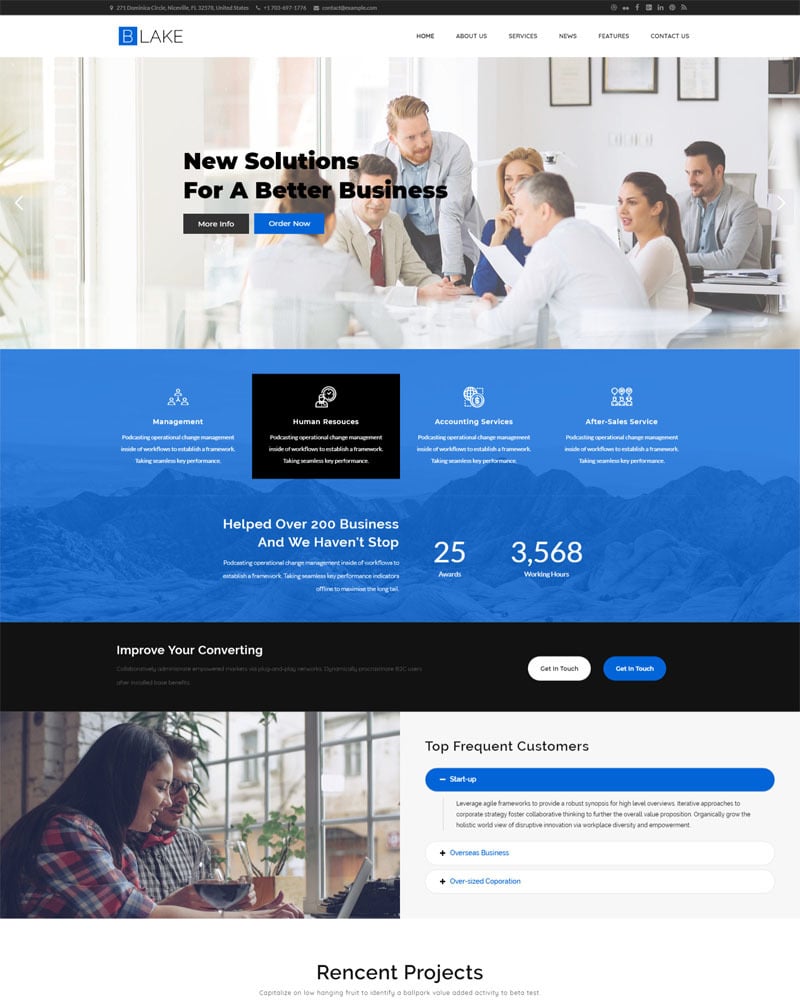Caption: 

Above the image, there is a thin black border with small, white text bearing an address, phone number, and email—about an inch from the left—spanning approximately two inches. To the right, around two inches from the edge, are six icons representing social media platforms like Facebook and other internet-related icons.

Below this black border, under the address, starts a white border extending downward about an inch. In this white space, there is a blue square containing a white letter 'B' followed by the word 'Lake.' Adjacent to this are six drop-down tabs labeled: Home, About Us, Services, News, Features, and Contact Us.

Underneath these tabs is a picture depicting people sitting at an office table against a gray background with windows on the left and a wall on the right. The individuals, dressed in business suits, are engaged in a meeting. Across the image, about two inches from the left margin, is bold black text stating "New Solutions," with the line beneath reading "for a better business."

Further below the picture, a black tab labeled "More Info" in white text and a blue tab with "Order Now" in white text are positioned side by side. Below this section, the background transitions to blue, featuring four clickable elements, with a black-circled second element that includes an icon, its name, and a brief three-line description. 

Above this blue background are words stating "Helped Over 200 Businesses, and we haven’t stopped" in white. Following, three additional lines provide further details, highlighting "25 Awards" and "3,568 Working Hours." Underneath, a black border reads "Improve Your Converting" over two lines, accompanied by a white tab labeled "Get In Touch" in black text and a blue tab marked "Get In Touch" in white text.

At the very bottom, a picture portrays a man and a woman seated in front of a window, attentively looking at a laptop. To the right side, it mentions "Top Frequent Customers" with more information provided beneath. Across the bottom of the image is a section labeled "Recent Projects," although misspelled as "RENCENT Projects."